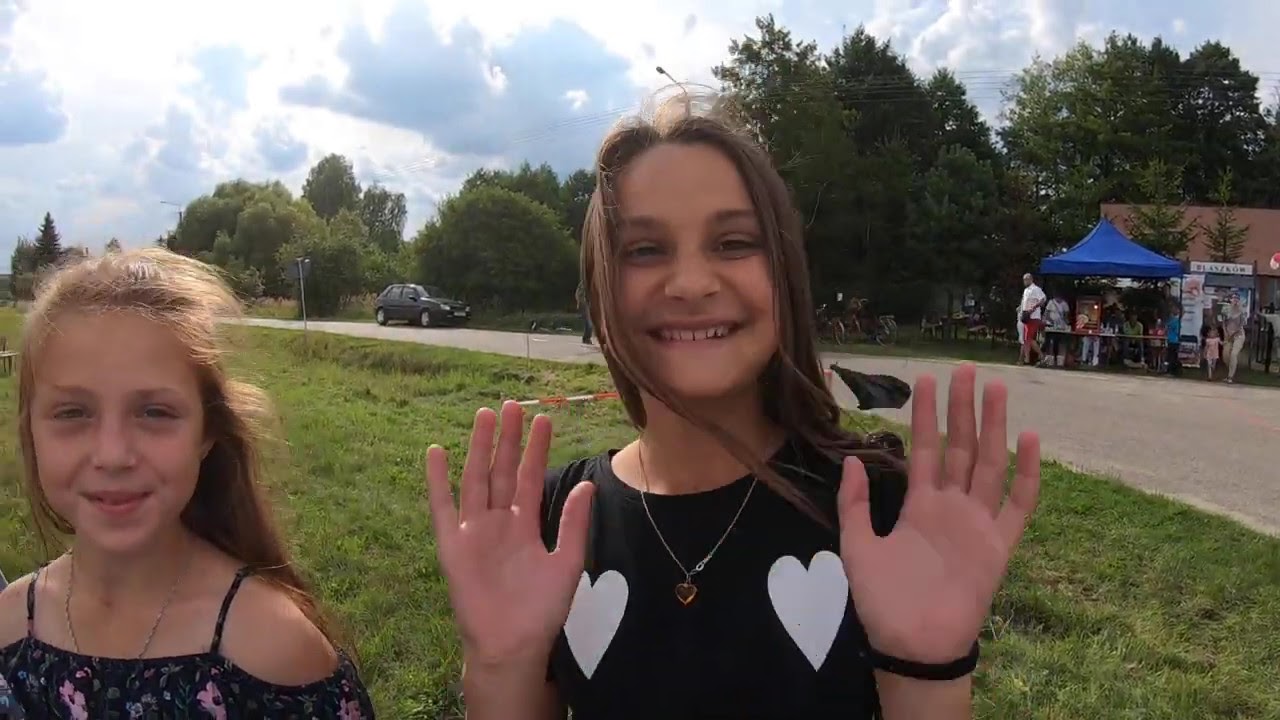This color photograph, in a landscape orientation, features two young girls standing outdoors and smiling directly at the camera. The central girl, approximately 15 years old, has long brown hair and is wearing a black shirt adorned with two white heart designs—one on each side of her chest. She is also wearing a small necklace and has both of her hands raised with her palms facing the viewer. To her right, there is a younger girl, around 12 years old, with long brown hair and a strappy dark blue top decorated with pink flowers. Both girls are Caucasian and smiling warmly. 

In the background, there is a grassy field leading to a curved gray asphalt road with a gray sedan parked along it. Towards the right side of the image, a small stand with a blue canopy is visible, where several people appear to be gathered. The surrounding scenery includes tall green trees, a blue sky, and numerous fluffy white clouds, creating a pleasant and sunny daytime atmosphere. This photorealistic image captures a lively and natural outdoor moment.